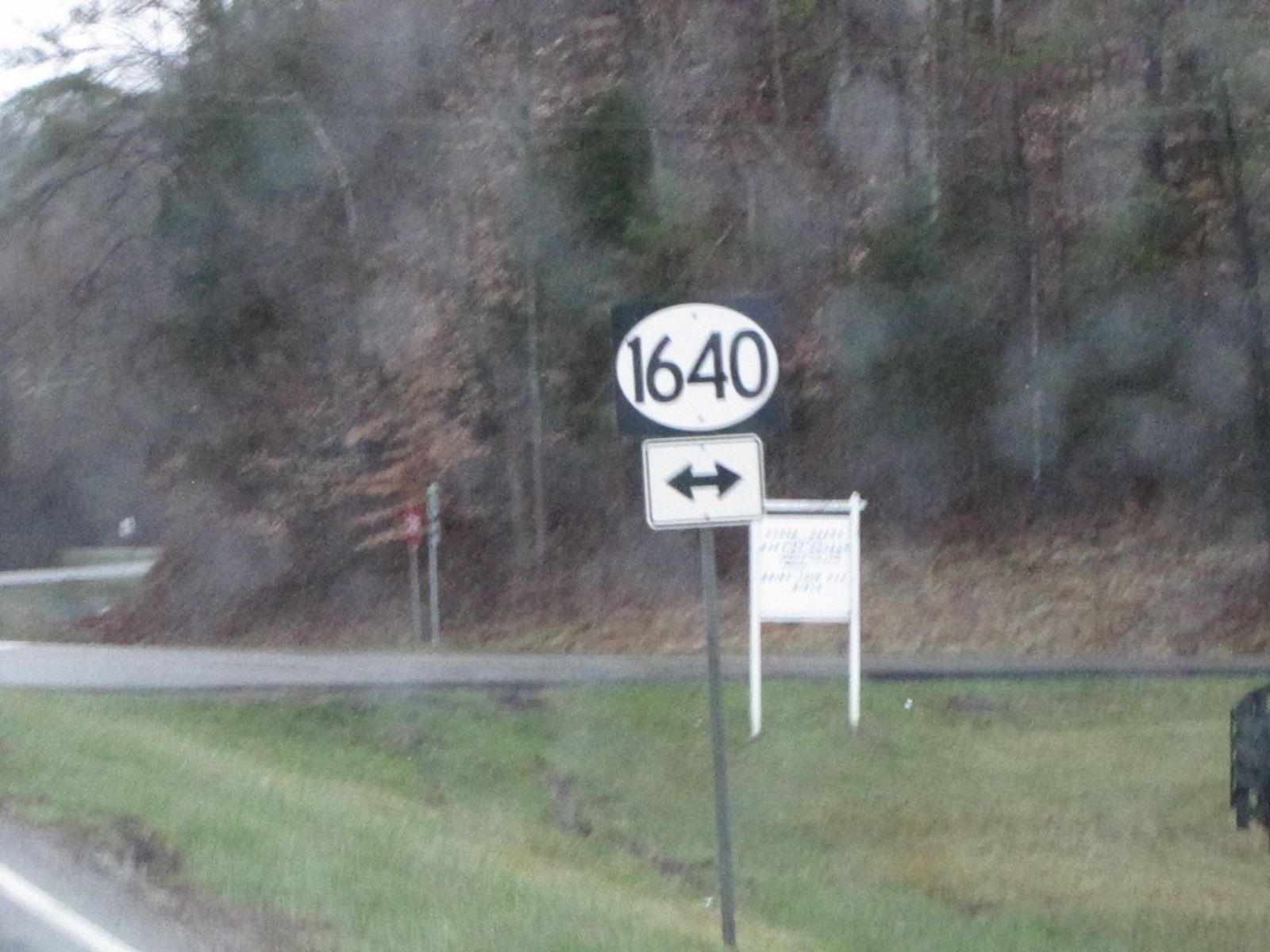This roadside photograph, taken from inside a moving car, captures a slightly blurry and foggy scene, indicative of the contrasting temperatures between the cold outside and the warm inside of the vehicle. Dominating the image is an oval road sign displaying the number '1640,' positioned above a pair of arrows pointing left and right, guiding travelers to their respective directions. In the background, partially obscured yet visible, is what appears to be a 'For Sale' sign, adorned with some writing and set against a backdrop of tall, towering pine trees. The road in the foreground intersects with another road, presumably the one designated as 1640, drawing the viewer's eye toward the dense woods that add a sense of depth and seclusion to the photograph.